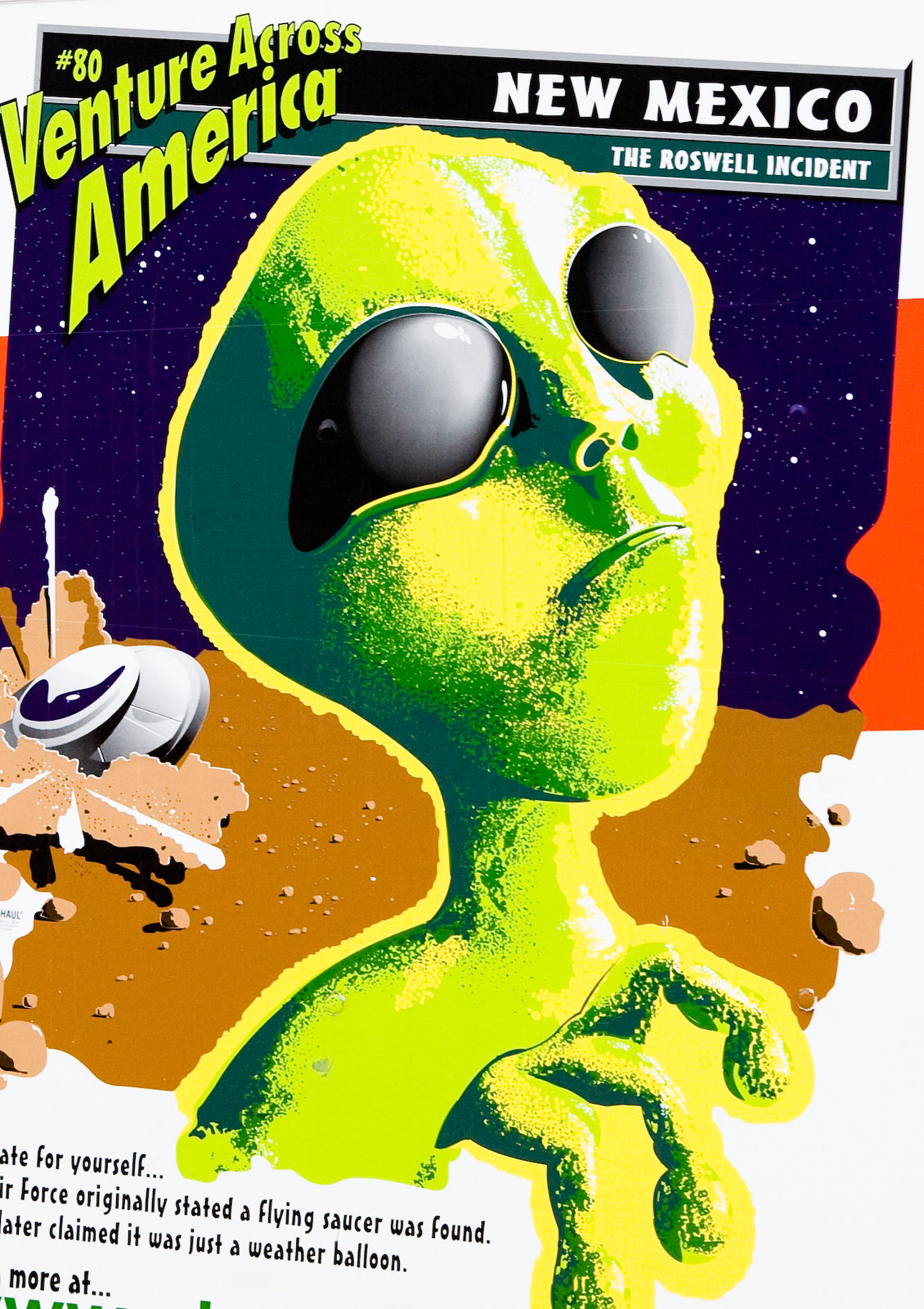The image is a vibrant and detailed cover, likely for a magazine or book, with a focus on the Roswell incident. Dominating the center is a green alien with a slender frame, a teardrop-shaped head, large black eyes, tiny nostrils, and only three fingers per hand. The alien appears to be looking up towards the starry blue sky, depicted with white dots to simulate space. Positioned near the top left, in bright lime green, is the text "Venture Across America," accompanied by the number 80 in the same color. To the top right, in white text, it reads "New Mexico, the Roswell incident." Below this, there's a depiction of the alien's surroundings—a desert landscape filled with sand and rocks, further emphasizing the crash site of a flying saucer located to the left of the alien. The bottom part of the image has a white background with black text that's partially cut off, making it difficult to read in full but hinting at a narrative: "Force originally stated a flying saucer was found. Later claimed it was just a weather balloon." The overall style is somewhat cartoony, with elements designed to draw in the viewer's eye to the dramatic, extraterrestrial scene.